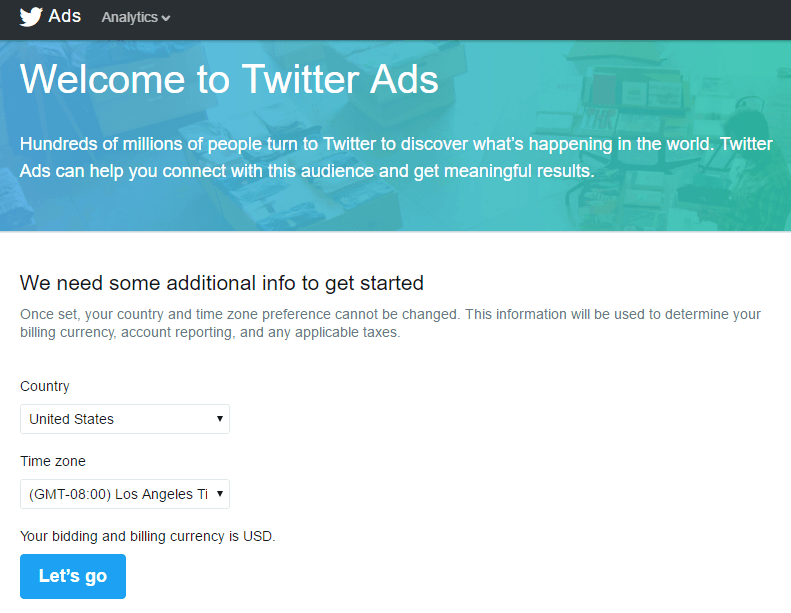The image showcases a Twitter interface designed for advertisers. At the top of the display, there are two tabs labeled "Twitter" and "Ads," followed by another tab titled "Analytics." Below this section, a large blue bar prominently features the text "Welcome to Twitter Ads" in white lettering. The accompanying message reads, "Hundreds of millions of people turn to Twitter to discover what's happening in the world. Twitter Ads can help you connect with the audience and get meaningful results. We need some additional info to get started. Once set, your country and time zone preference cannot be changed. This information will be used to determine your billing currency, account reporting, and any applicable taxes."

Further down, the interface shows a country selection drop-down menu with the United States pre-selected, though the other options are not visible. Similarly, there is a time zone selection menu showing "GMT-8:00 Los Angeles time" as the selected option, with no other choices displayed. The chosen billing currency is listed as USD. At the bottom of the display, a button labeled "Let's go" invites the user to proceed.